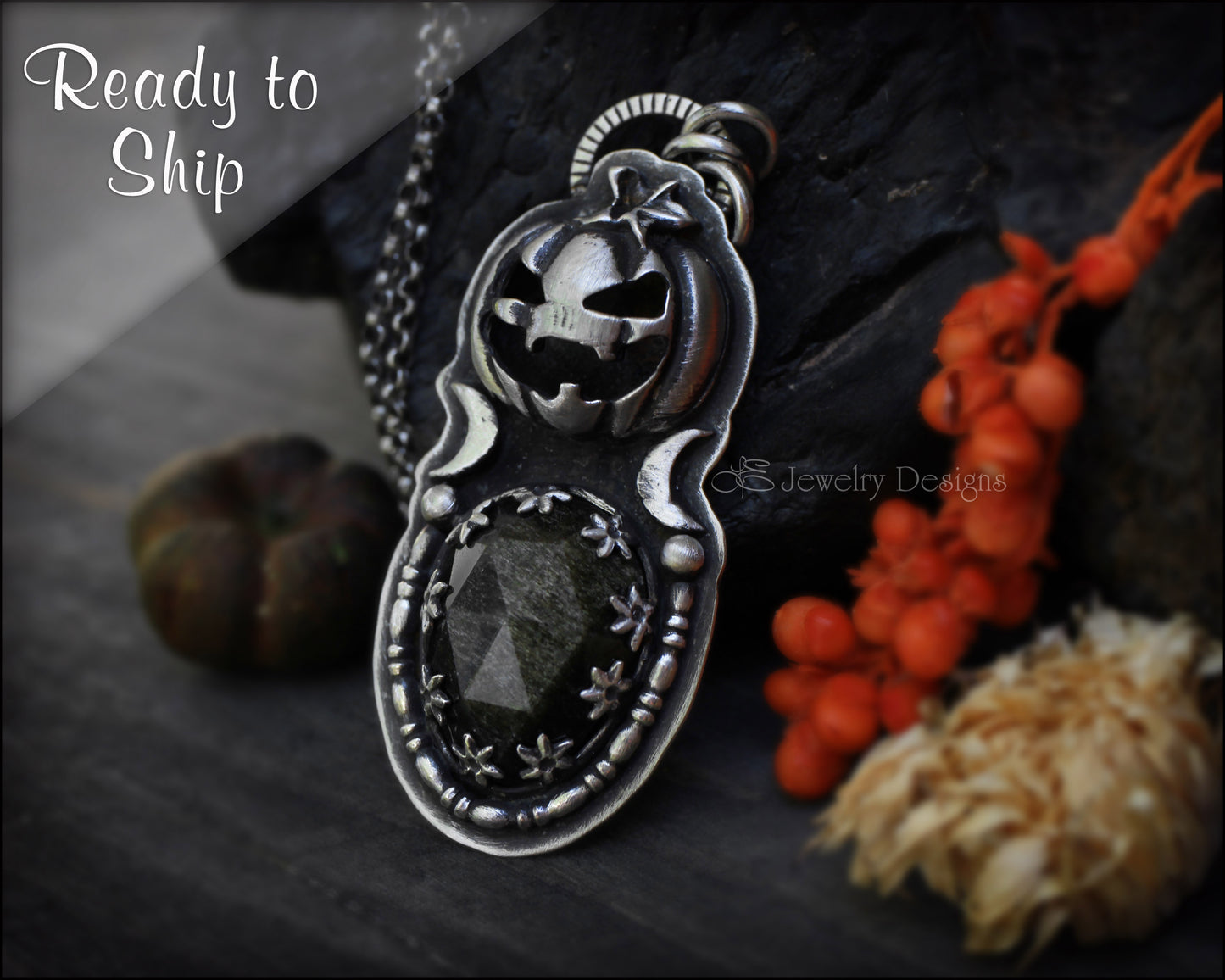The image showcases a meticulously detailed, silver-colored necklace laying against a backdrop of dark gray wooden texture. Central to the necklace design is a striking jack-o'-lantern with an evilish grin, positioned at the top. Below the jack-o'-lantern, two crescent moons elegantly flank a pendant that features a dark, ruby-shaped stone adorned with intricate silver flowers. The pendant itself is framed by a horseshoe-like metal outline and connected to a sophisticated silver chain with a pattern of scattered cylinders. Positioned on the left side of the image is a small black pumpkin, while to the right, red berries and a pile of tan wheat provide a complementary, organic touch. The entire ensemble rests against some black fabric, creating a dramatic contrast. The frame includes text reading "ready to ship" at the top left, and additional jewelry designs are visible nearby, enhancing the overall theme of artisanal craftsmanship.